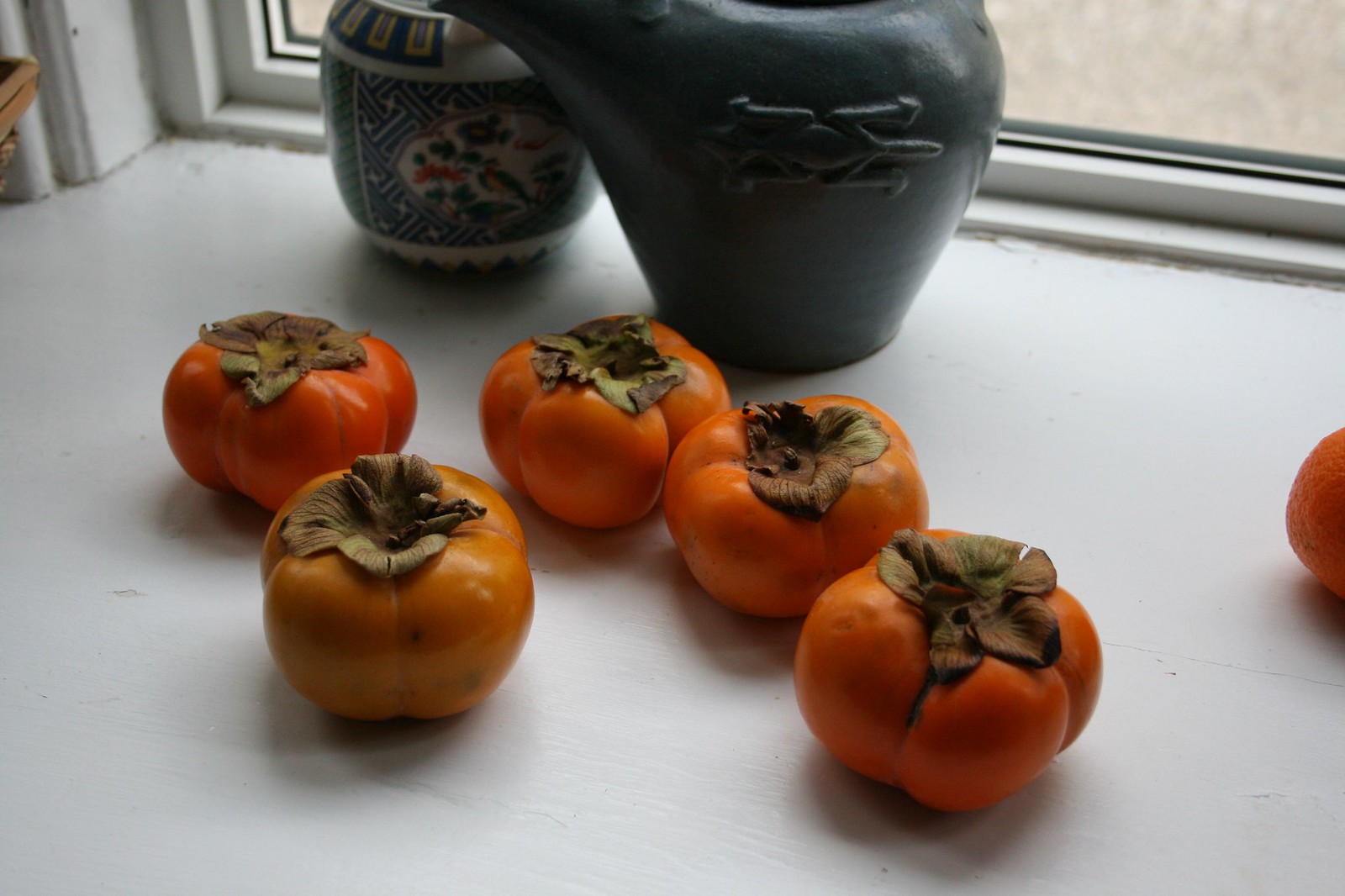A close-up, color photograph features five deep orange to light orange tomatoes, likely homegrown and possibly heirloom due to their unusual shape with four distinct sections and cross-like indentations. Arranged on a white countersill, three tomatoes are centrally positioned while two sit on the left. Adding another touch of color, an additional partly visible orangish fruit is located off to the right. A leaf, browning at the edges, crowns one of the tomatoes, indicating where it was plucked from the vine. The backdrop includes a green plastic watering can with its spout extending out of view at the top center, and to its left, a ceramic cup adorned with a blue gardening design. The setting appears to be a windowsill, likely on a cloudy day, given the faint light filtering through a possibly visible window or wall.